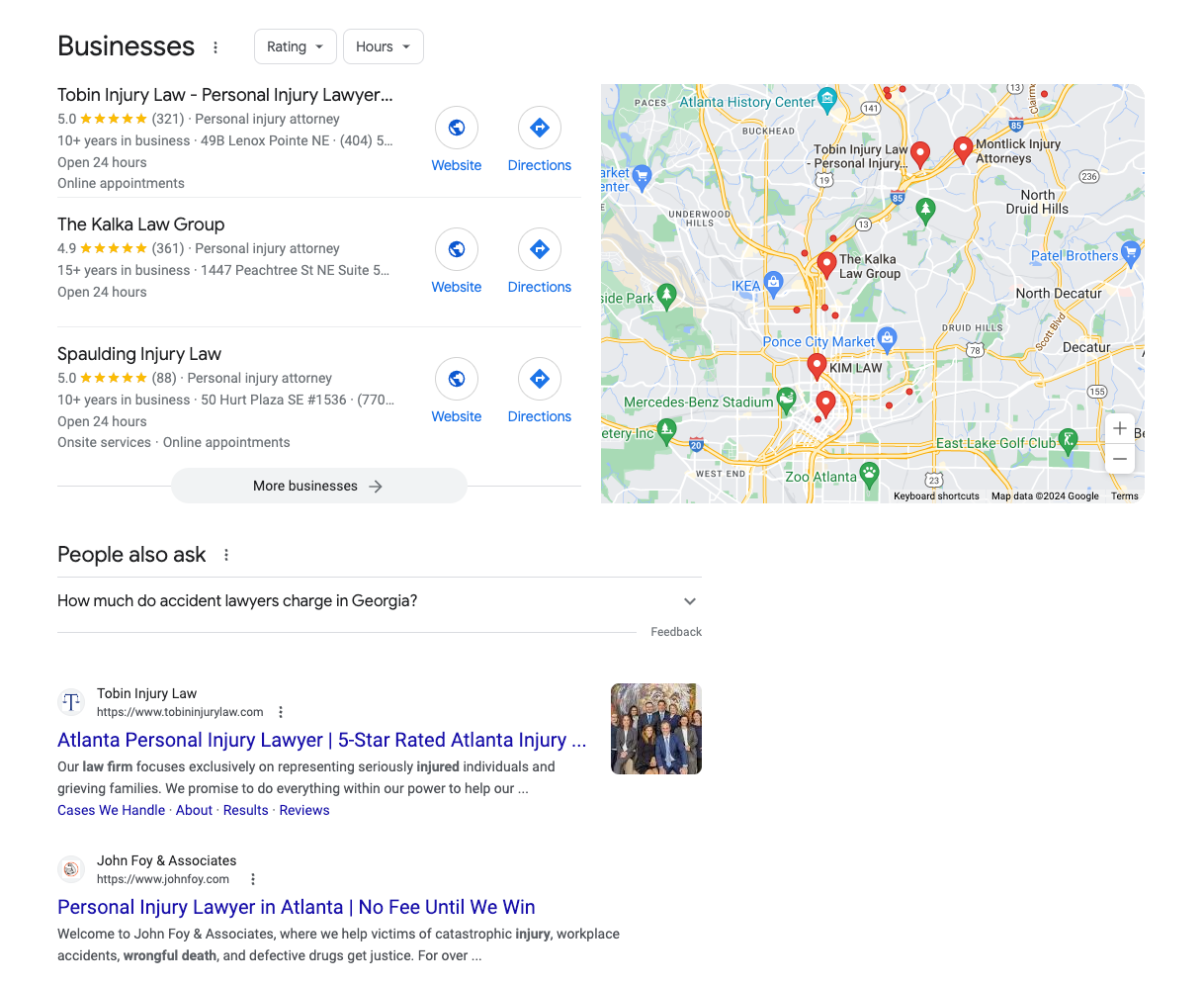In this image, set against a solid white background, we see a screenshot. On the right side of the image, there is a map from Google Maps showing the area around Atlanta, Georgia. Atlanta is positioned in the upper left corner of the map, with surrounding areas including Wood Hills and Buckhead below it, and North Druid Hills and North Decatur to the east.

To the left of the map, there is a list of businesses presented in bold black text. The first listed business is "Tobin Injury Law," identified as a personal injury lawyer. This listing features a five-star rating in yellow stars and has 321 reviews indicated beneath it. To the right of this entry are action buttons in blue text and circles; the first button labeled "Website," followed by another labeled "Directions."

Following Tobin Injury Law in the search results are two other law firms: "The Kalka Law Group," and "Spalding Injury Law." Each of these listings follows the format of the first, though specific details such as reviews and ratings are not mentioned. The overall presentation is clear and organized, providing a thorough overview of personal injury law firms in the Atlanta vicinity.